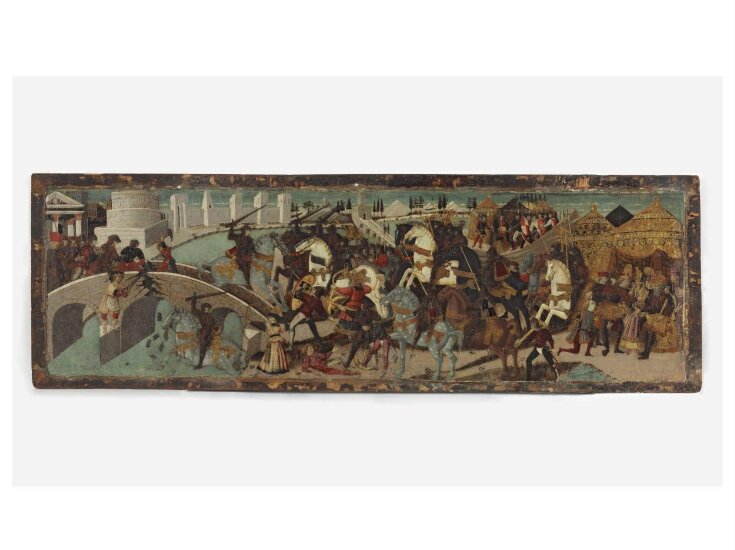The artwork is a sprawling horizontal painting, approximately five feet by two feet, depicting a chaotic battle scene from ancient times. Its style appears to be Byzantine, with a distinctly antiquated aesthetic that suggests it could be a genuine antique or a skillful replica. The painting is possibly rendered on a medium like clay or wood, hinted by its cohesive outer edge. The image's details are intricate yet somewhat blurred, primarily showcasing a tumultuous war scene filled with warriors brandishing swords, bows, and arrows. Some figures are mounted on horses of varying colors—brown, gray, white, and black—that are either engaged in combat or bucking amidst the chaos.

The background appears to include depictions of water, although it's somewhat ambiguous due to the painting's busy nature. There are old structures and buildings, with notable features like gold huts in the right corner and a small bridge with soldiers crossing it on the left side. These soldiers are on foot, contrasting with the mounted ones, and adding to the complex layering of the battlefield. The palette consists of pale tones of gold, sea green, tan, and dark red, set against a light white backdrop, which creates a nuanced and somewhat ethereal depiction of this dramatic historical warfare. Details such as columned buildings evoke a sense of ancient Greek or Roman architecture, enhancing the painting's historical aura.